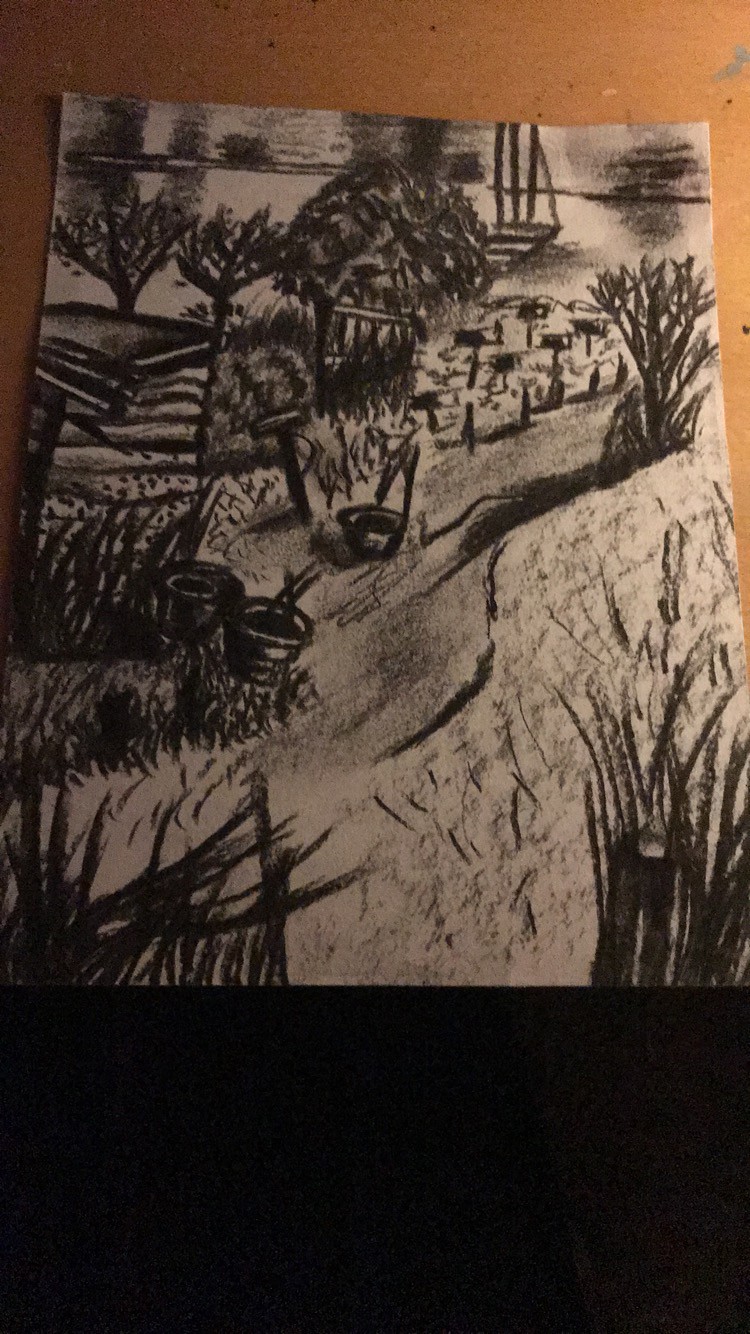The image presents a detailed pencil drawing on white paper, set against a tan or cork-like background with a visible tack at the top right corner. Depicted in rich graphite or charcoal, possibly black pastel, the black-and-white sketch foregrounds a meandering dirt path starting from the bottom left, curving gently leftwards before veering right and continuing off the image. This path leads through a grassy field dotted with tufts of longer grass, especially on the right side. To the left, several flower pots and baskets are scattered on the ground, hinting at a pastoral farm scene. Large tufts of grass are interspersed throughout the field, adding texture. In the top center of the drawing, a cluster of mature trees stands, beneath which small wooden structures are visible. The backdrop suggests the presence of water, discernible through subtle shading that creates a reflective effect, completing this serene rural tableau.